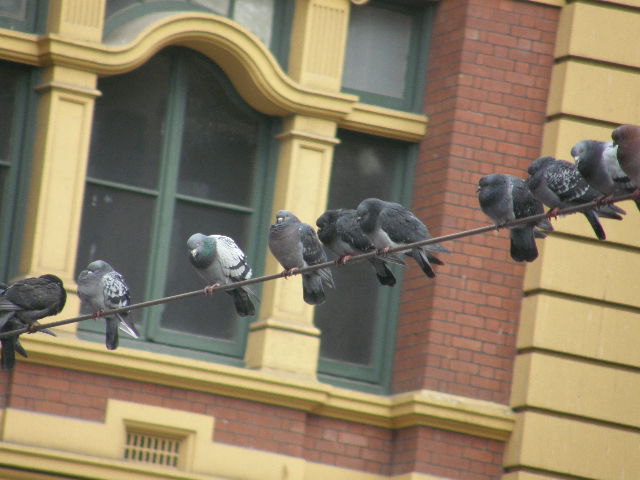The photograph showcases a group of 10 pigeons comfortably perched on a telephone wire, set against the backdrop of a high-rise building. The building features a mix of architectural details: the right side displays cream-colored building blocks, while the left side showcases brown brick with yellow siding around the windows. The large, curved windows are black, framed in dark green, and additional yellow trim can be seen, particularly near an air vent at the bottom. The pigeons, which appear to be mostly dark gray with a few sporting light green feathers and black beaks, are arranged along the wire, each puffing up their chests and mostly looking towards the ground. One pigeon stands out with a primarily white underside and wings marked by two black stripes, while the others are uniformly dark gray with occasional patches of brown. The scene gives a comfortable, cityscape vibe with its detailed urban setting and resting birds.